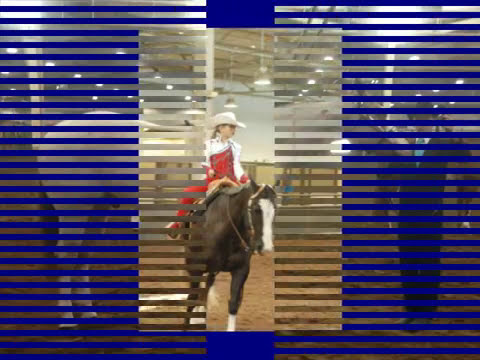In this detailed image, a young girl, approximately 10 years old, is portrayed riding a dark brown horse with distinctive white markings—a white stripe running down its face and white fur around its ankles. The girl, wearing a white long-sleeve shirt under red overalls, paired with a white cowboy hat, embodies the essence of a young cowgirl, possibly participating in an equestrian class or a barrel racing contest. Her blonde hair peeks out from beneath her hat. The horse is equipped with a rust-colored saddle and stands or runs on a dirt or sand surface inside an arena. Background details include blue horizontal lines and the faint image of a white horse and a figure of a man in a dark suit with a hat. The arena is well-lit from the ceiling above, indicating an indoor setting, likely captured on a smartphone due to the aspect ratio and quality of the image.